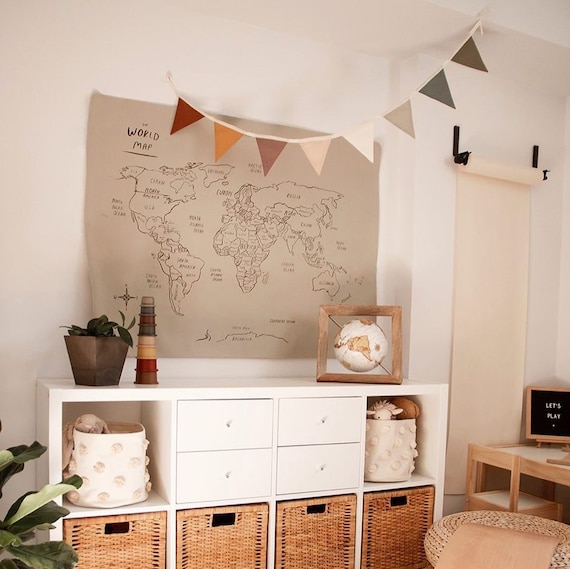The photograph showcases a child's bedroom, viewed at an angle that provides a detailed look at one side of the room. The focal point is a large, off-white to beige wall adorned with a world map. This map, in subdued earth tones of brown, highlights the continents and oceans with fine black outlines and labels. Above the map, a handmade banner featuring triangles in shades of red, brown, beige, orange, and gray hangs from the white ceiling.

Below the map, a white cubby shelf stands prominently. It contains four square wicker baskets in the bottom row and four rectangular white drawers in the middle. The open shelves flanking these drawers contain white, beige, and polka-dotted fabric bins, adding to the organized yet decorative appearance. On top of this shelf, on the left, there is a potted plant with lush green leaves, and to the right, a beige and white globe with a wooden frame is positioned at an angle.

To the right of the shelf, partially obscured by the angle, sits a white desk accompanied by a small brown chair. On the desk, there's a black chalkboard sign displaying the words "Let's Play." Behind this setup, a long roll of what appears to be burlap or paper is visible, adding a touch of rustic decor to the room.

Overall, the image encapsulates a cozy and educational playroom with ample storage, decorative elements, and a gentle, earthy color palette.